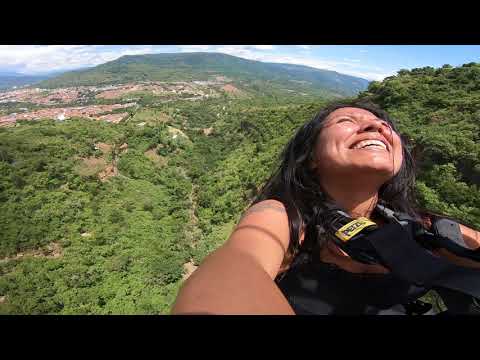A vibrant photograph captures a woman in the right third of the frame, her long dark hair cascading as she looks up at the sky with a joyful, wide smile. She is wearing a sleeveless black harness adorned with a yellow tag that reads "Petzl," indicative of climbing or other outdoor adventure gear. The woman’s arms are bare, suggesting she is in athletic attire, possibly a tank top. The photograph is taken from a slightly elevated angle, emphasizing that she is high up, likely suspended on a bungee or climbing, given her positioning and gear. Below her, a lush, green expanse of trees blankets the terrain, interspersed with valleys and small settlements in the distance. The backdrop features a majestic mountain range and a partly cloudy blue sky, enhancing the adventurous and exhilarating mood of the scene. The image itself is framed by long black bars running horizontally along the top and bottom, adding a dramatic effect to this thrilling capture.